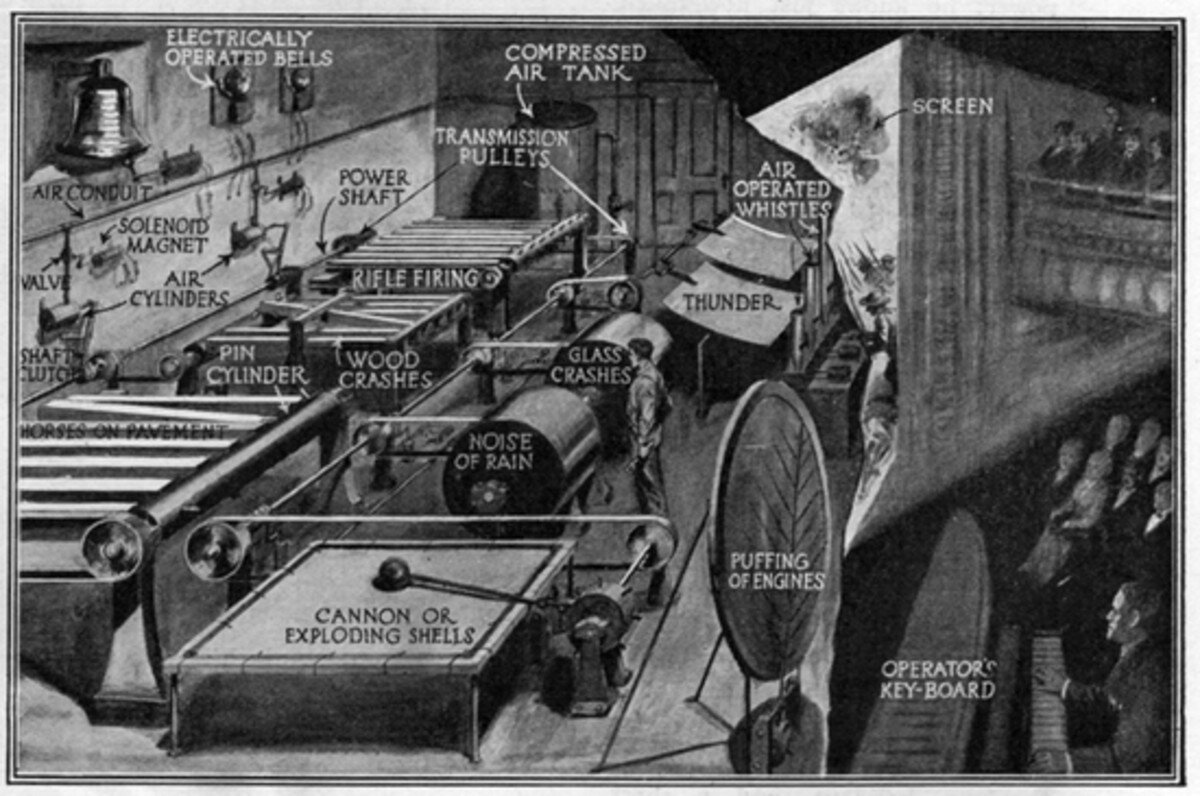The illustration, rendered in realistic black and white pencil, captures a behind-the-scenes look at a sound effects setup for a stage production. The detailed drawing, which appears to be from the late 1800s or early 1900s, showcases an array of complex machinery and their associated sound effects. 

On the left side of the image, various sound-producing contraptions are meticulously labeled. At the top is a "Compressed Air Tank," with additional components like "Transmission Pulleys," "Power Shaft," "Rifle Firing," "Wood Crashes," "Pin Cylinder," and "Horses on Pavement" following below. Specific sound effects such as "Noise of Rain," "Glass Crashes," "Air-Operated Whistles," "Thunder," "Puffing of Engines," and "Cannon or Exploding Shells" are also labeled, indicating their source mechanisms. 

Against the wall are "Electrically Operated Bells," "Magnets," "Air Cylinders," and "Air Conduit," adding to the intricate system of sound creation. Toward the far right side, the scene shifts to an audience seated in a theater, with sections identified for both upper gallery and lower level viewers. 

In the bottom right corner, a key figure operates a large labeled "Operator's Keyboard," signifying the control center for the various sound effects. The setup is visually connected to a "Screen" that the audience is viewing, bringing the scene's auditory elements to life.

Overall, the illustration serves as an informational chart detailing the elaborate orchestration of sound effects in a historical theater setting.